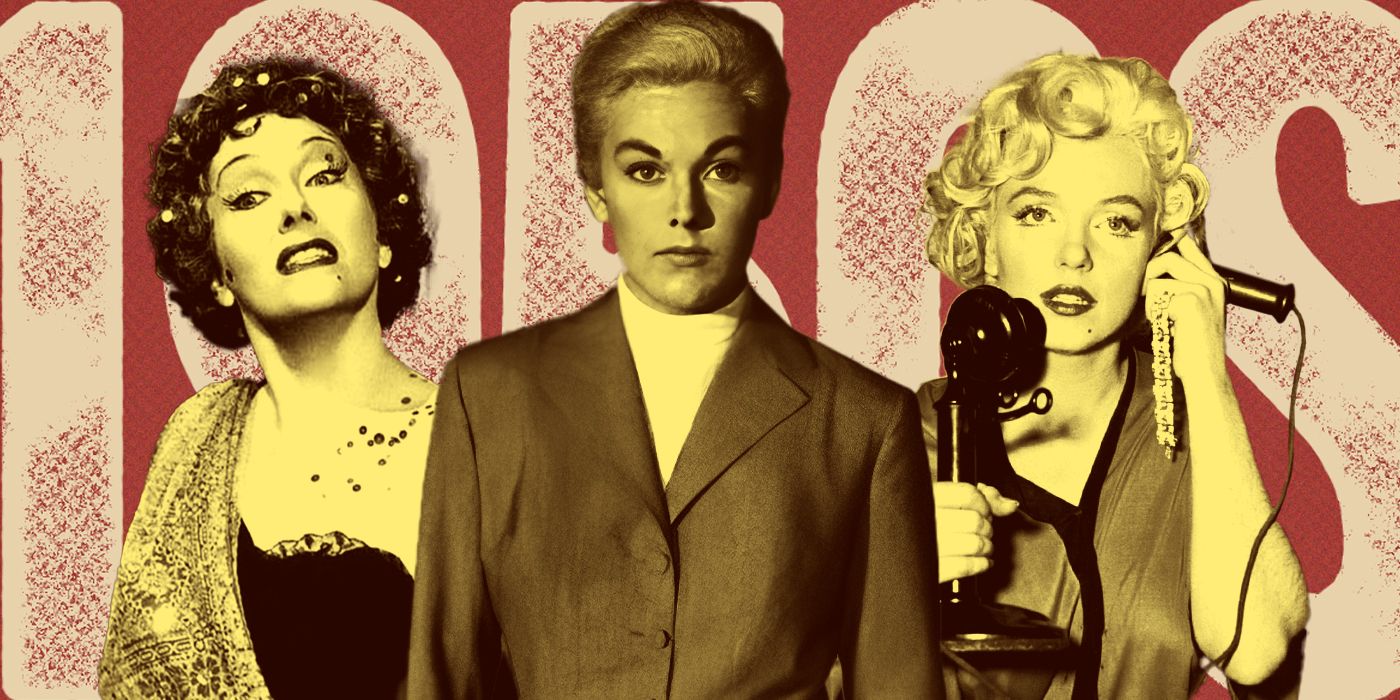The image is a black-and-white poster featuring three women, reminiscent of actresses from the 1950s. Against a red background with a large, stamped "1950s" in white font, the women are spotlighted in a compelling collage. On the left is a woman with curly black hair adorned with hair pieces, wearing a strapless black dress accented with a scarf draped over her left shoulder. She has heavy makeup, including winged eyeliner and black lipstick, and looks upwards with her chin raised. In the center stands another woman with short, polished hair and dark, prominent eyebrows. She wears a white mock neck shirt paired with a plain, dark blazer. Her expression is serious as she looks out directly into the audience. On the right, a woman with curly blonde hair, reminiscent of Marilyn Monroe, holds a vintage old-fashioned telephone with her left hand to her ear. She is dressed in a robe with a black border and is heavily made up with lipstick. The blend of these distinct personas captures a nostalgic essence of 1950s glamour and elegance.